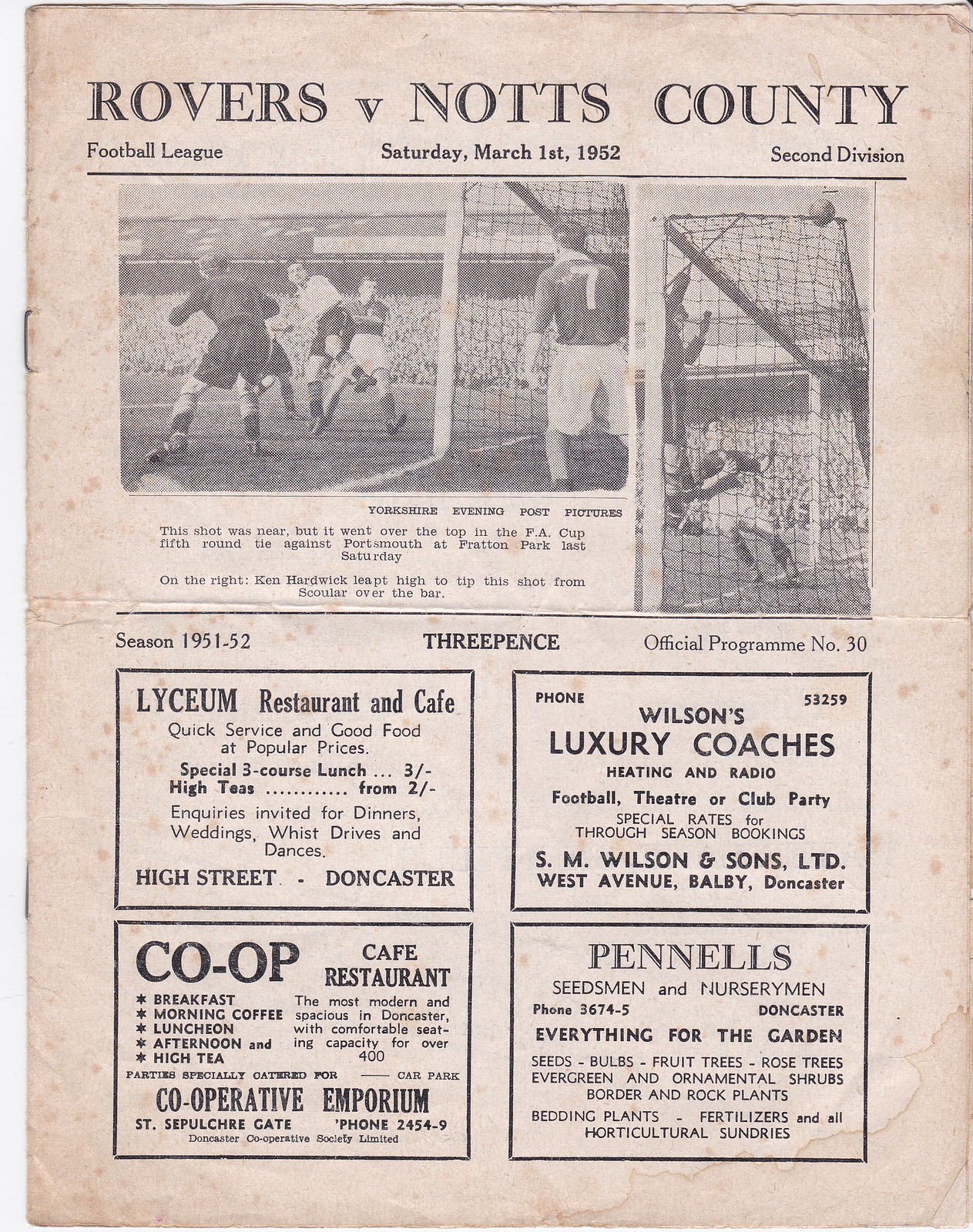The image depicts the front cover of a worn and stained soccer program from March 1st, 1952, for a Football League 2nd Division match between the Rovers and Knott's County. The details and age of the document are evident in its spots, creases on the edges, and a notable stain at the bottom right corner. The top of the program prominently features the match details: "Rovers vs. Knott's County," followed by "Football League, Saturday, March 1st, 1952, 2nd Division," with "Season 1951-52, Three Pens, Official Program, Number 30" mentioned slightly below. The center section includes two black-and-white images of players engaged near the goal area, above a caption referring to a near-miss shot from an FA Cup fifth-round tie against Portsmouth at Pratton Park. The bottom half is divided into four advertisement rectangles: the upper left advertises the Lyceum Restaurant and Cafe offering quick service and good food, the upper right promotes Wilson's Luxury Coaches with heating and radio services, the lower left highlights the Co-op Cafe Restaurant known for its modern and spacious seating for over 400 people, and the lower right features Pennell's, Seedsmen and Nurserymen, catering to all garden needs. Two visible staples on the left binding attest to its age and use.